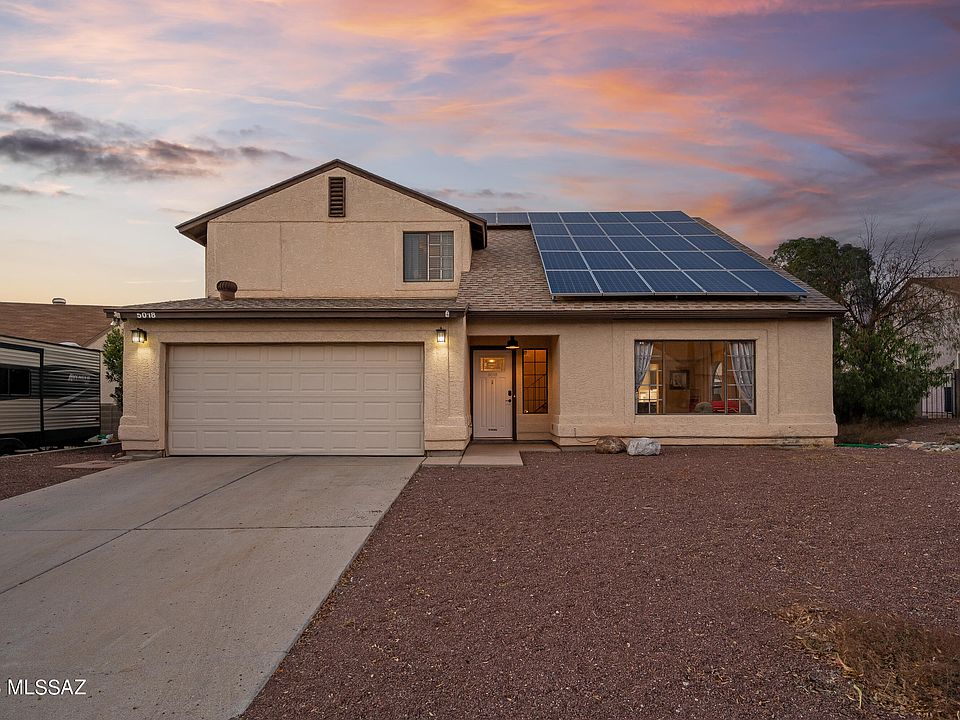Photograph of a tan-colored house likely listed on the Multiple Listing Service (MLSSAZ), featuring a double car garage on the left side. The garage is framed by light-colored brick pillars, each adorned with a wall-mounted sconce light. The house primarily features a single-story design, except for a second story situated above the garage. Interestingly, the second story has an asymmetrical appearance with a window on the right side and a boarded-up section, painted to match the siding, on the left.

The roof is covered with light brown shingles and heavily laden with solar panels that span approximately four-fifths of its surface. The front yard is xeriscaped with gravel and minimal plant life, save for a couple of trees on the right side, which may belong to this or a neighboring property.

At the time the photo was taken, it is sunset, as indicated by the illuminated sconce lights and the pendant light over the front door entry. The interior lights of the home are also visible. The neighboring property to the left has a large travel trailer RV parked in its driveway, partially visible in the photo.